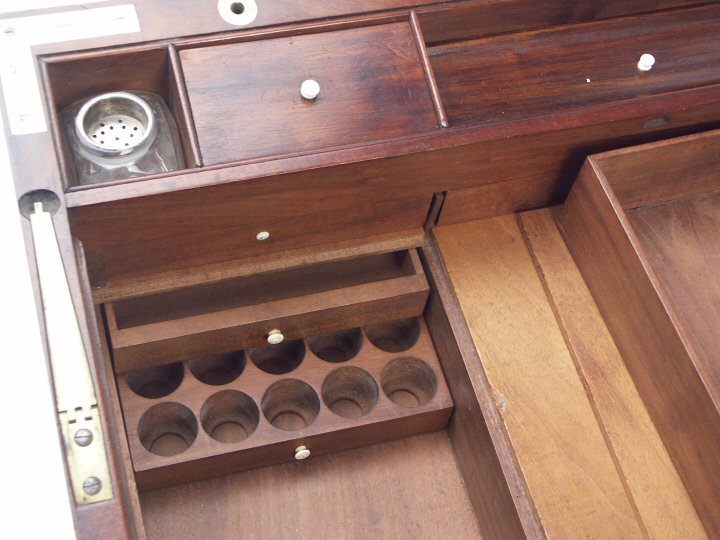The image showcases a rustic, dark cherry wooden cabinet or tackle box taking up the entirety of the frame, with no visible background. The furniture piece, which occupies a centered but slightly diagonal position, features various drawers and compartments hinting at multifunctional use, possibly as a kitchen, apothecary, or tea storage unit. Notable details include an assortment of small, white, round drawer pulls, and distinctive circular indentations visible in the bottom drawer meant for organizing or storing round objects. One particular drawer houses a small glass jar with a perforated white lid, resembling a mini shaker. The upper left corner of the image reveals a hollow, silver metal object, potentially part of the jar or a separate item with multiple holes. The overall color palette includes different shades of brown, tan, and accents of silver and white, with some light streaming in from the upper left, hinting at a nearby window. The setup, characterized by various sections and angles, adds a unique, somewhat disoriented charm to the piece, making it visually intriguing yet complex in design.